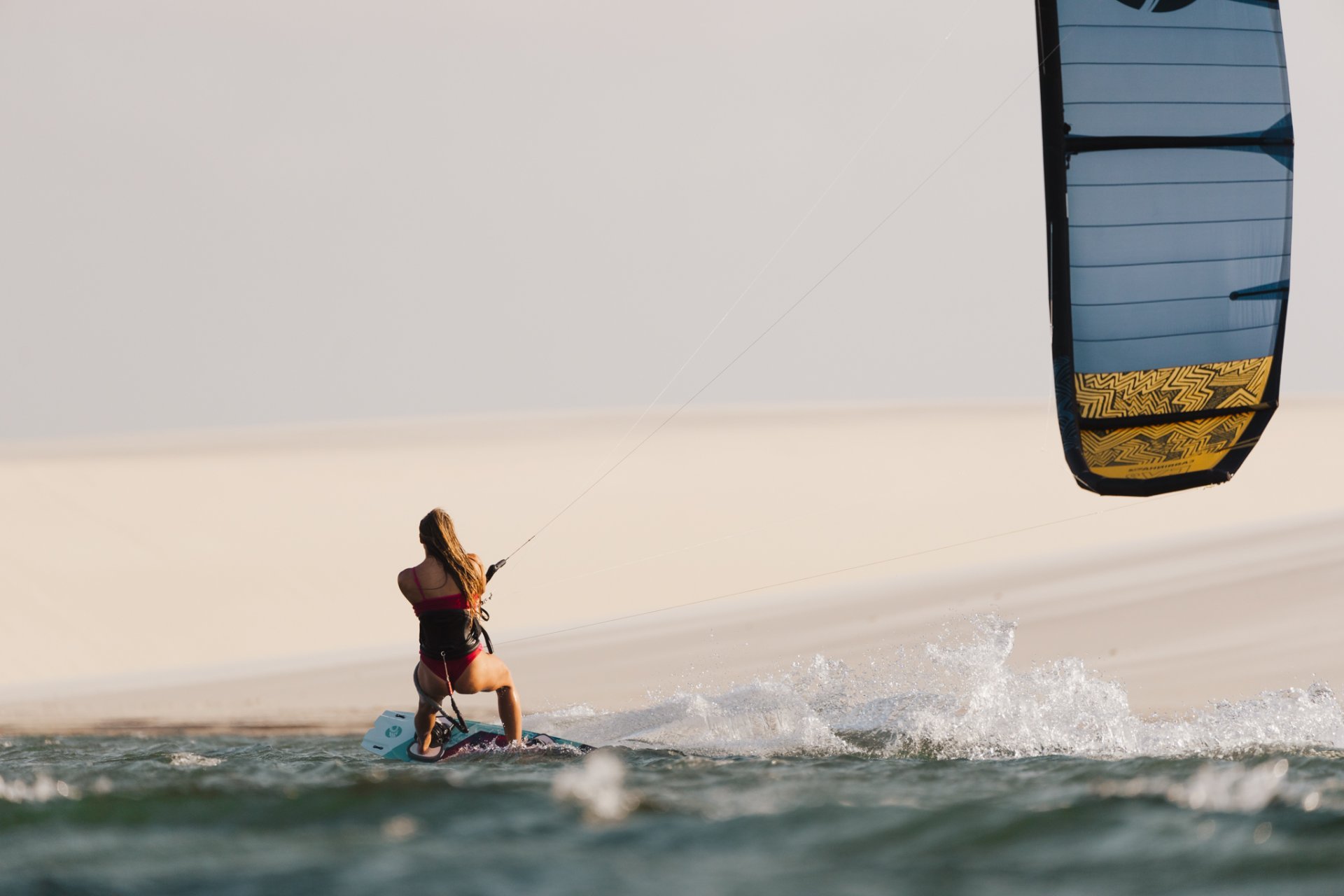In this captivating image, we see a woman kitesurfing on an ocean or large body of water. Her back is to the camera, revealing her long brown hair tied back in a ponytail. She is dressed in a red one-piece swimsuit, supplemented by a harness connecting her lower back to the surfboard. Her legs are muscular and bent at the knees as she balances on a white and blue surfboard, navigating through the dynamic, greenish-blue waves. The water splashes around her, indicating a windy day; brilliant white crests of waves contrast against the water's surface.

In her hands, she grips a handle attached to a blue and black striped kite, accentuated with yellow zigzag tribal patterns. This kite, featuring a highly reflective surface, seems to mirror the sandy beach in the distance or perhaps it's just an intricate pattern. The kite is positioned in the upper right part of the frame, with the woman situated toward the lower-middle left. The sky above is partly cloudy with streaks of white against a hazy blue backdrop, enhancing the scene's sense of motion and energy. The meticulous composition of the image beautifully captures the thrill and intensity of kitesurfing.